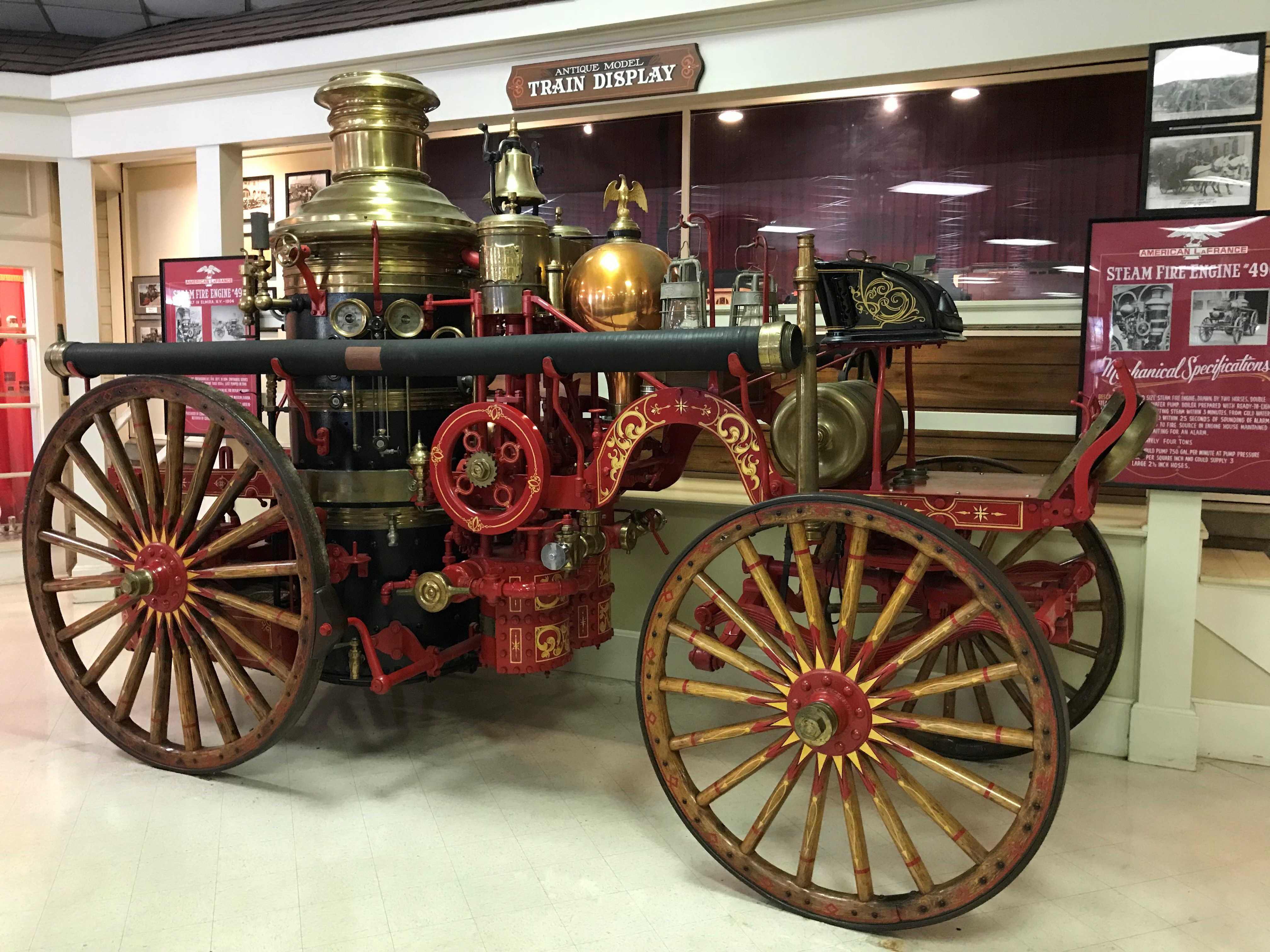The image captures an antique model train display within a train or transportation museum, prominently labeled as such by a sign at the top center of the photo. Dominating the scene, the model showcases an early 1900s steam fire engine, distinguished by its intricate details and vibrant colors. The steam fire engine, marked as "Steam Fire Engine 49," features four large wooden wheels with yellow and red accents reminiscent of suns. The engine is adorned with elaborate gold and red accents, especially on the wheels and pipes, while the main body is painted in red and gold, complemented by black sections. Notably, a majestic gold eagle perches atop the model train. The machine exudes an old-timey charm with its dials, handles, and connecting pipes, accentuated by multiple pressure gauges. The back displays a prominent black and bronze steam engine, complete with a singular pipe, bronze cylinders, and spherical elements. At the front, small black benches situate themselves on a flat red platform, ready for the driver. Against the backdrop of the museum, with additional signage and pictures, the display sits next to a window, making the historic marvel even more eye-catching.